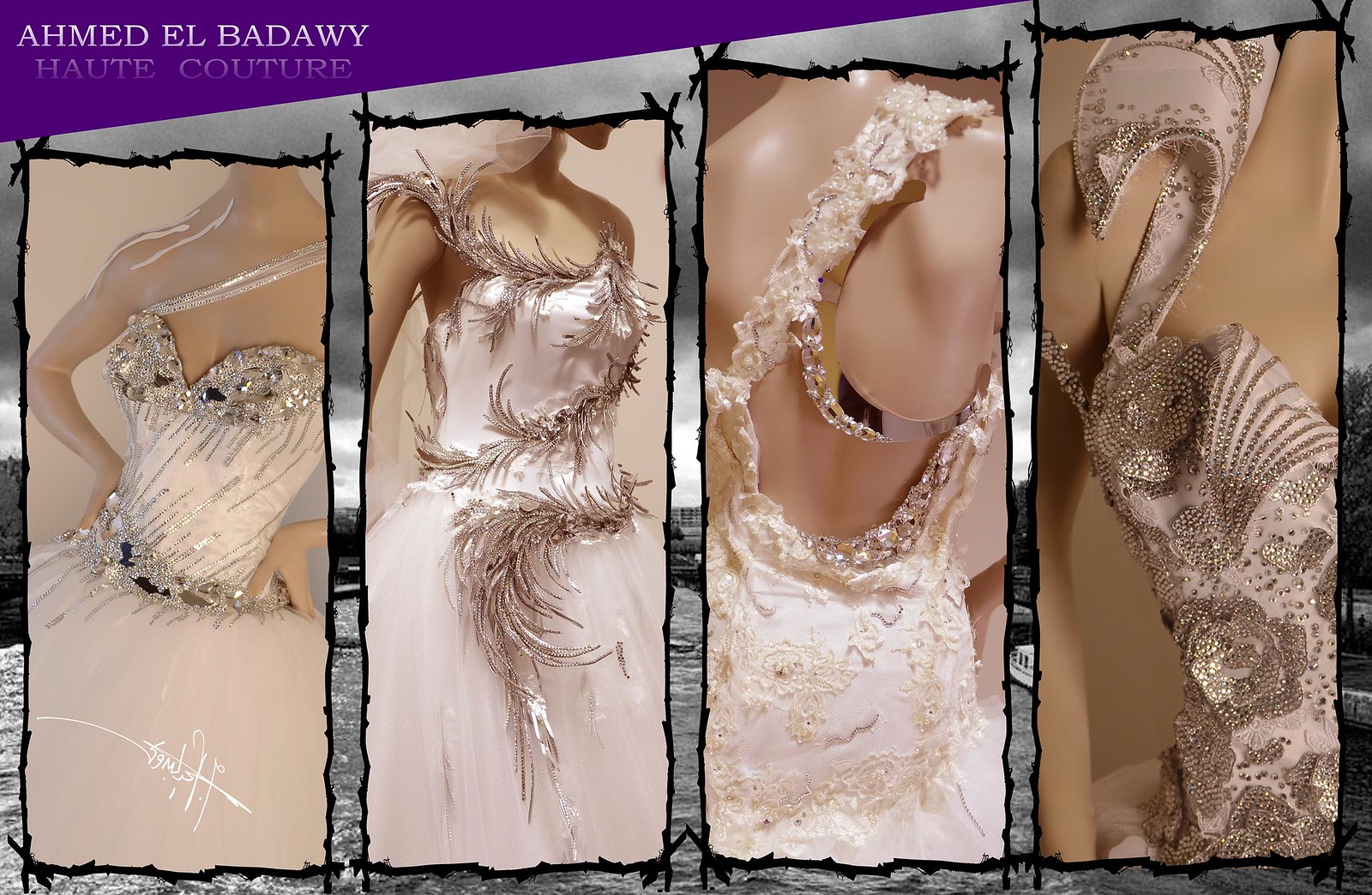The advertisement showcases four detailed, close-up photographs of mannequins adorned in elaborate white and silver bridal gowns. The dresses, designed by Ahmed El Badawi and labeled under "Haute Couture," feature intricate silver embellishments in various styles, including silver detailing on the chest, neck, and back. These photographs are arranged in a row against a greyish, black and white background which is difficult to discern but seems to depict a blurred cityscape or river scene. In the top left corner of the image, a slanted purple triangle contains the designer's name and collection title. The overall composition presents a sophisticated and glamorous selection of bridal wear, emphasizing the luxurious details of each gown.